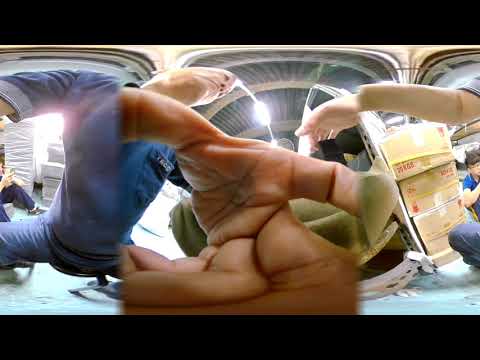The image depicts an Asian man around 40 years old, sitting on the floor, wearing a blue t-shirt and blue jeans. The central focus of the picture is his open hand, prominently zoomed in, showing the palm with the thumb and index finger up and the other fingers curling down. The image has a strong distorted effect reminiscent of a funhouse mirror or 360-degree imaging, which warps and elongates the features. The man's head and body are similarly distorted.

To the left side of the image, you can see part of the man's body distorted, with his torso elongated and limbs shortened. In the background, there appears to be another person squatting. On the right, there is an arm—possibly dislocated due to the effect—and boxes that look like they are tilting inward. There are also several workers, some appearing to be carrying stock, and what looks like a green chair and a dolly with stacked boxes. The floor appears blue and there are three archways in light brown.

The photo has black bands framing the top and bottom, adding to its surreal appearance. This combination of extreme close-up and heavy distortion makes the scene look as if viewed through a funhouse mirror, emphasizing the hand in the center while blurring and warping the surrounding environment.